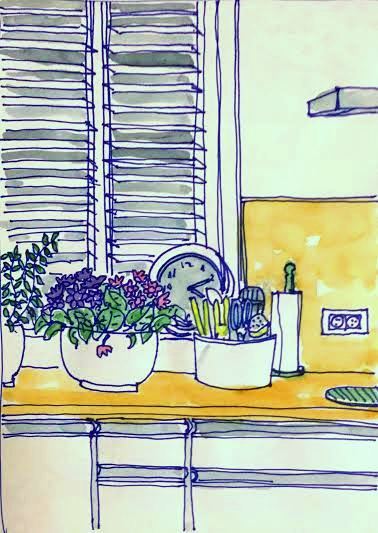This illustration depicts the interior of a kitchen, skillfully rendered using a combination of watercolors and possibly markers. Dominating the scene is a golden yellow countertop and matching backsplash. On the top left corner of the image, a window with vertical slats, resembling Venetian blinds, features a white frame and two rows of slats. Propped on the bottom right corner of the window sill is a clock, displaying the time as ten past four, although part of its face is obscured by a white container filled with various kitchen tools, including a pair of blue scissors. Adjacent to this is a green paper towel holder with a roll of paper towels. Below the counter are white cabinets and drawers, highlighted with a distinctive blue outline, adding a touch of artistic flair to the scene. Additionally, there are two white pot holders on the left side of the image: one houses green leaves with purple and pink flowers, while the other, partially cut off, contains a vine-like plant with small green leaves. An electrical outlet is visible on the backsplash completing this detailed and vibrant kitchen illustration.